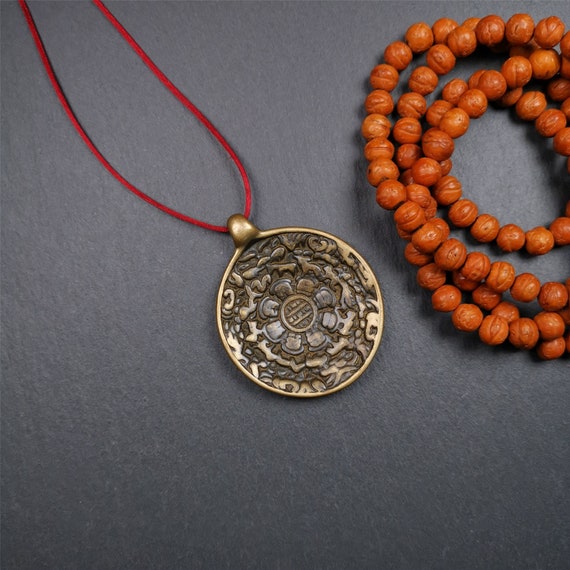The photograph captures two distinct necklaces resting on a dark gray background, possibly a countertop or table. Centrally positioned is a necklace featuring a red string that supports a round, intricately engraved golden medallion, resembling an antique coin with detailed squiggly lines and a floral pattern of petals encircling a central circle. This medallion appears to have small perforations in its intricate design. To the right, a long necklace composed of wooden beads, predominantly orange in color with tiny faint black markings, is coiled in a circular shape. The image solely focuses on these two pieces of jewelry against the muted backdrop, emphasizing their contrasting yet complementary designs.